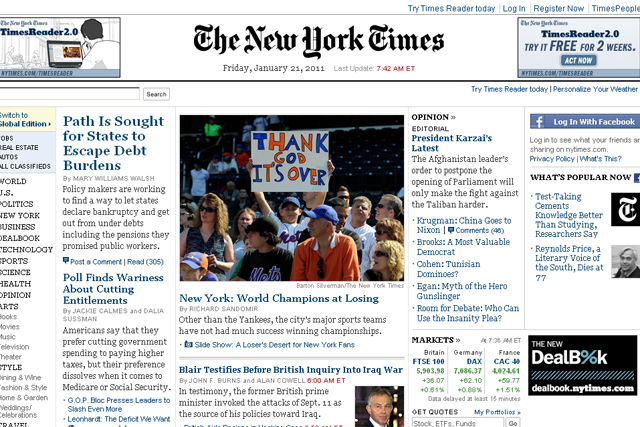### Detailed Description of The New York Times Web Page Screenshot

In this detailed screenshot of The New York Times web page, the prominent masthead features "The New York Times" in its iconic black, cursive font. Directly below this, the date is displayed as Friday, January 21st, 2011, in a light black, standard Arial font. Notably, the latest update time, 7:42 a.m. Eastern Time (ET), is highlighted in red for easy visibility.

On the left side of the page, there is an advertisement for "Times Reader 2.0," showcasing an animated drawing of a person using a laptop. This ad is mirrored on the right side of the page, promoting a free two-week trial of the "Times Reader 2.0."

Below the masthead and advertisements, there is a search bar labeled "Search" on the left side. To the right of the search bar, there is additional promotional text: "Try Times Reader today. Personalize your weather."

Continuing down the page, a series of articles are presented. The most prominent feature is a central picture of a young boy dressed in a white baseball jersey with the word "Mets" emblazoned across it. He is wearing a baseball cap and holding up a handwritten sign in multiple colors, stating, "Thank God it's over." The letters on the sign alternate between blue and orange, and the crowd around him is seated with some empty seats visible in the background.

Below this central image, there is an article titled "New York: World Champions at Losing," authored by Richard Sandomir. Another article directly beneath is titled "Blair Testifies: British Inquiry Into Iraq War," featuring a picture of then-Prime Minister Tony Blair.

To the left of this main article section are two additional articles: "Path Is Sought for States to Escape Debt Burdens," followed by "Poll Finds Wariness About Cutting Entitlements."

On the right side of the central picture, the Opinion page features an editorial titled "President Karzai's Latest," with a list of subsequent articles including topics like "China Goes to Nixon" and "Cuban and Tunisian Dominoes."

Further down, a Market Report section displays information on various stock indexes, including the DAX in Germany, as well as indices for Britain and France. On the far right, there is an interactive element inviting readers to "Log in with Facebook," presented in a blue bar. Underneath, there is a "What's Popular Now" section listing two popular articles and another advertisement for "DealBook" at the bottom of the page.

The far left shows a truncated view of more articles, indicating the page does expand further with additional content.